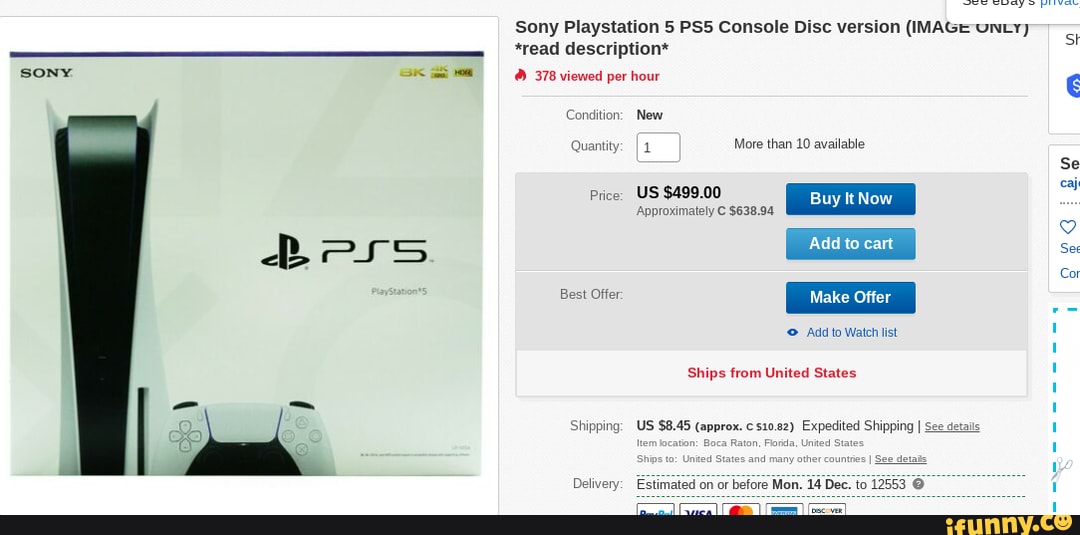The image prominently features the Sony PlayStation 5 (PS5) console against a white background, emphasizing its sleek design. On the left side of the image, the white casing of the PS5 is showcased, complementing its black interior. The console's DualSense controller also makes an appearance, featuring a predominantly white exterior with black shoulder buttons and a back accent. The controller's face displays the iconic PlayStation buttons: triangle, square, circle, and X.

The text within the image highlights the console's specifications and availability: it is the disc version of the PS5, priced at approximately $499 USD. The seller is located in Boca Raton, Florida, USA, and offers shipping to various countries, with expedited shipping options available within the United States for $8.45. The item is described as being in 'Neo' condition, with more than 10 units available for purchase. Interested buyers can choose to purchase directly, or make an offer, with options to add the item to their cart or watch list. The delivery estimate projects arrival on or before Monday, specified between dates 12/5 to 14/7.

Additional text visible in the image includes: "8K", "4K HDR", "Sony PlayStation 5", "PS5 console", "disc version", "read description", "view power", "condition", "quantity 1", "buy now", "add to car", "best offer", "make offer", "add to watch list", "ships from United States by Texas shipping," and "delivery estimate on and before Monday."